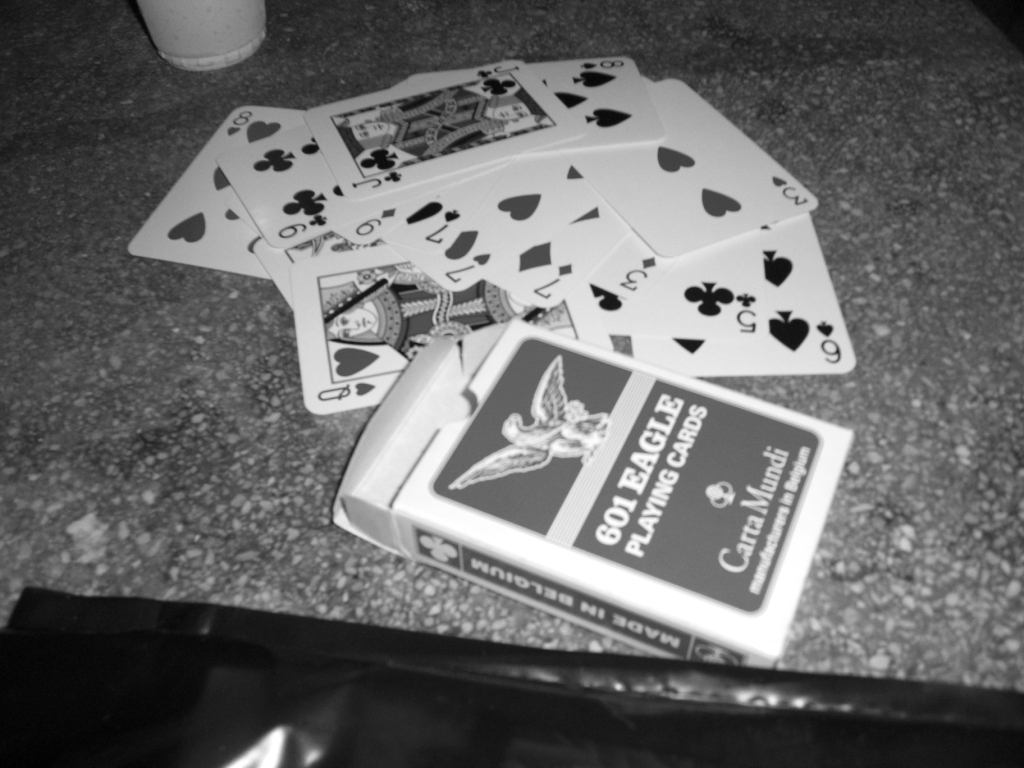This black and white image captures a close-up scene on a kitchen-like granite work surface, characterized by its speckled stone texture. Dominating the foreground is a reflective black plastic bag, occupying the bottom portion of the photograph. Just above the bag, you can see the work surface extending upward, partially obscuring the lower part of a plastic cup that is situated at the top edge of the image.

The central focus of the photo is a scattered assortment of playing cards and their empty packaging. The box, prominently featuring an illustration of an eagle and labeled with "601 Eagle Playing Cards, Carta Mundi," indicates that they were manufactured in Belgium, a detail reiterated on the side of the box. Approximately 10 to 15 cards are strewn across the work surface, adjacent to the box, suggesting that the entire deck might not be present. This disarray adds a dynamic element to the otherwise still life composition.